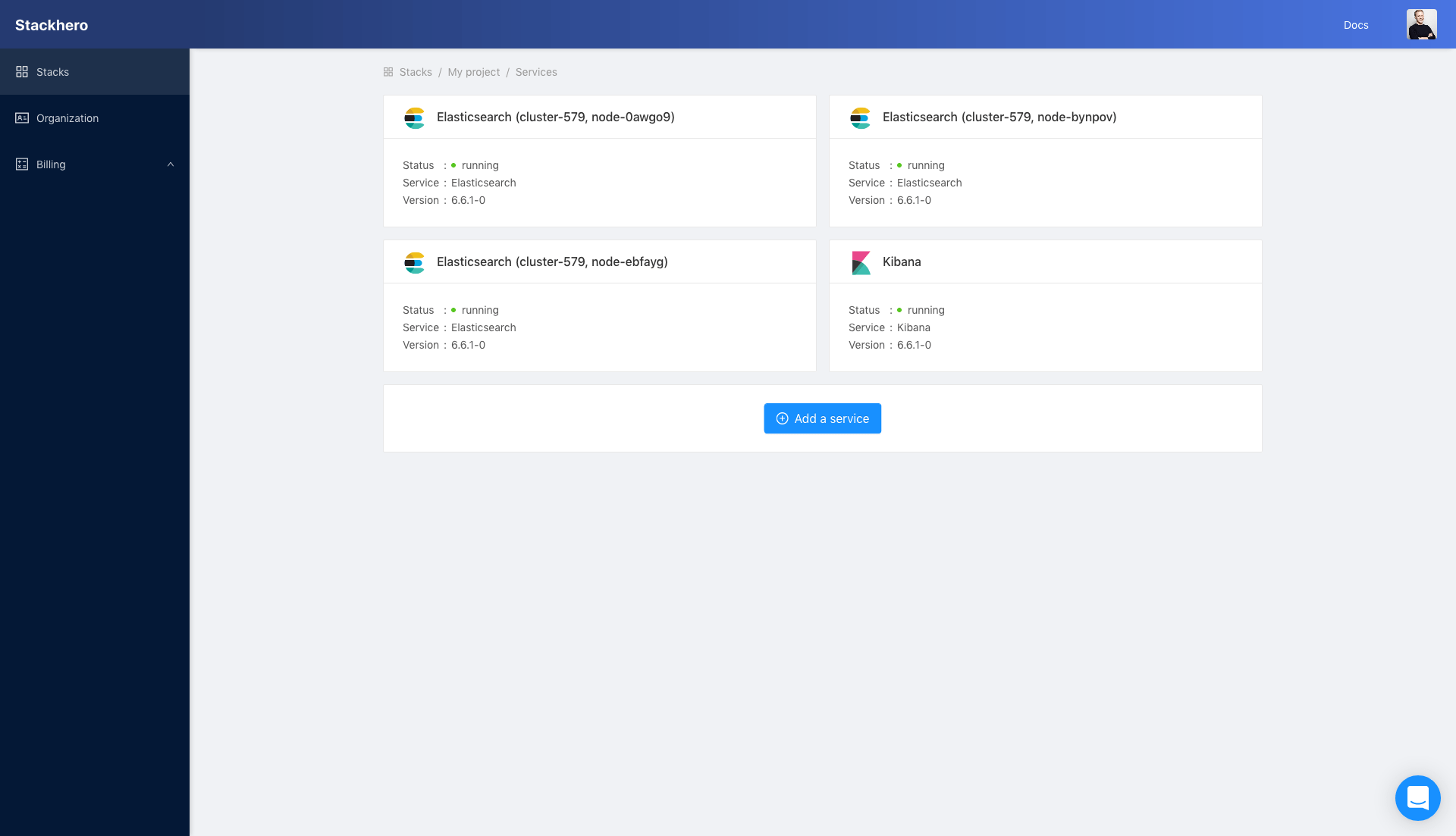The image depicts a detailed dashboard overview. 

At the very top, there is a prominently displayed stock hero image. Moving to the right side, there is an image labeled "Docs" showing a person folding their arms, wearing a jacket, against a white background. On the left side, there are sections labeled "Stacks," "Organization," and "Billing," with the "Billing" section highlighted in blue.

Centering the image, it shows navigation text: "Stacks / My Product / Services." Below this navigation path, there are detailed descriptions of several Elasticsearch clusters and services: 

- **Elasticsearch Cluster - 579**: 
    - **Node 0** (ID: AWG09): Status is running; Service is Elasticsearch, version 6.6.1-0.
    - **Node 1** (ID: BPOB): Status is running; Service is Elasticsearch, version 6.6.1-0.
    - **Node 2** (ID: EBFAyg): Status is running; Service is Elasticsearch, version 6.6.1-0.

- **Kibana**: Status is running; Service version 6.6-0.

There is also a mention of an "Added Service," but details are unspecified.

At the bottom right corner of the image, there is a distinctive blue circle icon.